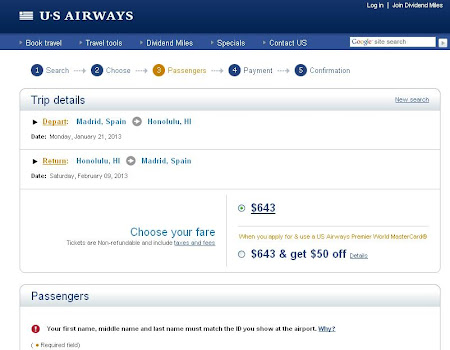This image is a screenshot of the U.S. Airways website interface. At the top, the iconic American flag logo alongside the "U.S. Airways" branding is prominently displayed against a blue background. The website's main navigation menu features sections such as "Book Travel," "Travel Tools," "Dividend Miles," "Specials," and "Contact Us." To the right, a Google site search bar is visible.

The central feature of the page is a five-step booking process displayed horizontally:
1. Search
2. Choose
3. Passengers (highlighted in orange)
4. Payment
5. Confirmation

Below the steps, a "Trip Details" section outlines the following itinerary:
- Departure: Madrid, Spain to Honolulu, Hawaii on January 21, 2013
- Return: Honolulu, Hawaii to Madrid, Spain on February 9, 2013

An option to "Choose Your Fare" is presented, offering a fare of $643. Additionally, there's a promotion: by applying for and using a U.S. Airways Premier World MasterCard, travelers can receive $50 off, effectively reducing the fare to $593. A "Details" button accompanies this offer.

In the "Passenger" section beneath, the website prompts users that their first, middle, and last names must match the identification shown at the airport, indicating the next step in the online ticket purchasing process.